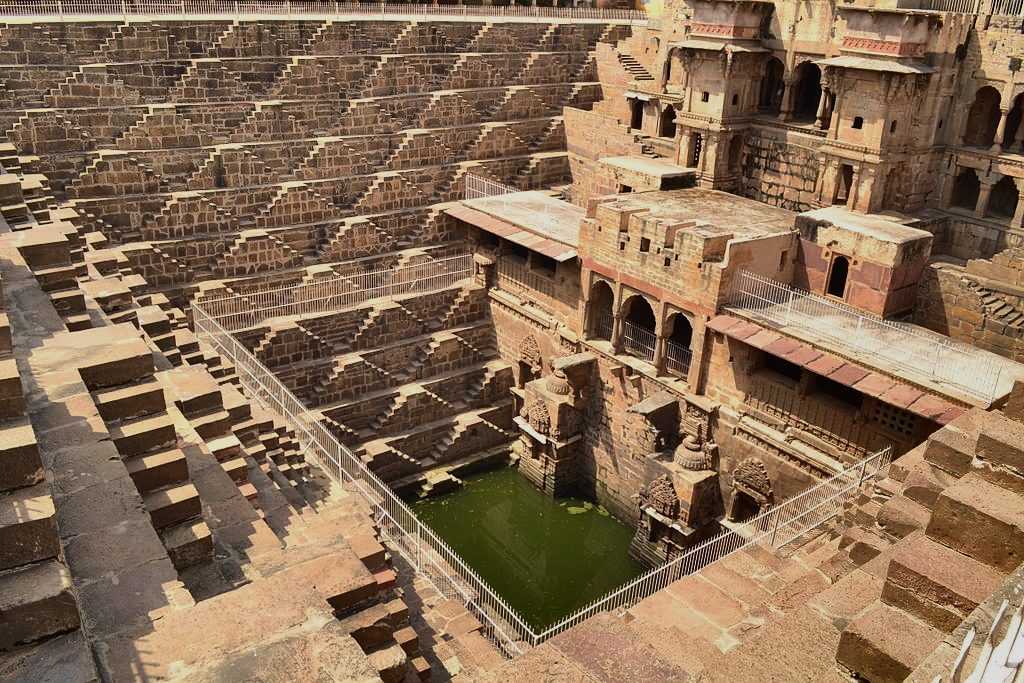The photograph depicts an ancient, vacant building complex with a magnificent architectural design in shades of tan and brown. The structure, largely made of stone, is arranged around a deep central courtyard containing a pool of murky green water. Notably, the courtyard is square-shaped and features many arched entryways, doorways, and alcoves. The levels within the courtyard rise on three sides, possibly serving as seating or steps, while the right side of the image reveals a more substantial building highlighted by ornate brickwork. The scene is fenced off with a white metal barrier, suggesting it might be part of a touring site or museum. The sunlight casts clear shadows across the photograph, adding to the sense of depth and antiquity.